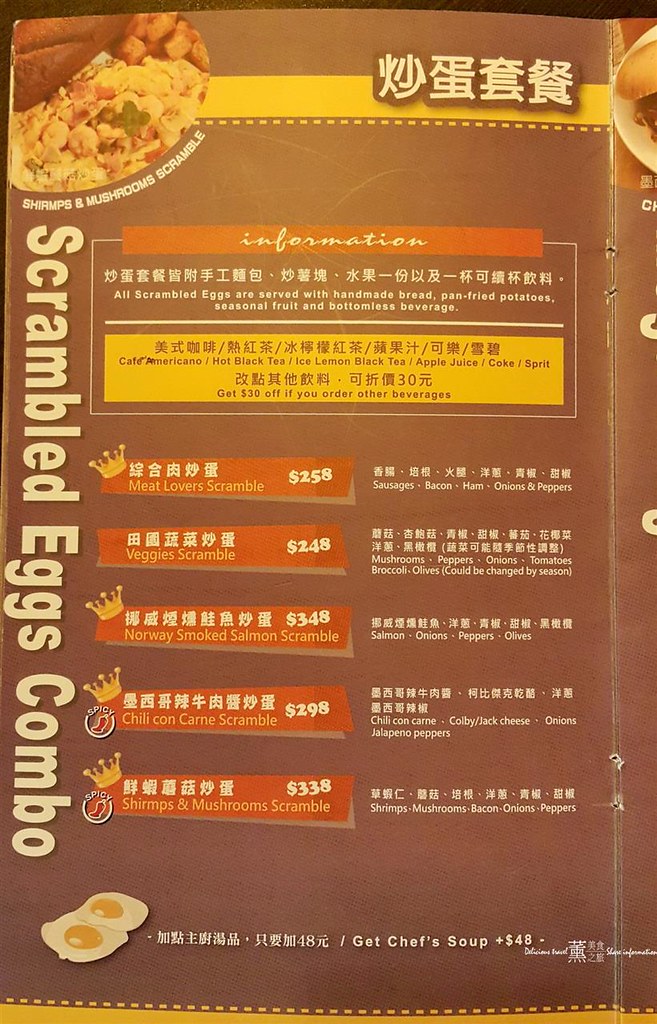**Restaurant Menu Description**

The menu presented features both English and Japanese text, designed against a basic brown background with a yellow and red color scheme for emphasis. 

In the upper left-hand corner, there is a photograph showcasing a dish comprising scrambled eggs with potatoes, labeled as "Shrimp and Mushrooms Scramble." 

Nearby, on the left-hand side, the section title "Scrambled Eggs Combo" is emblazoned in white lettering. 

A prominent yellow-bordered section at the top contains a red banner with the word "INFORMATION." Beneath this banner, it states: "All scrambled eggs are served with homemade bread, pan-fried potatoes, seasonal fruit, and bottomless beverage."

Following this, the yellow border details the available beverages: Café Americano, Hot Black Tea, Iced Lemon Black Tea, Apple Juice, Coke, and Sprite. It also notes: "Get $30 off if you order other beverages."

The main menu items are displayed within red banners, listing the offerings and prices:
- Meat Lovers Scramble – $2.58
- Veggie Scramble – $2.48
- Norway Smoked Salmon Scramble – $3.48
- Chili Con Carne Scramble – $2.98 (features a spicy logo)
- Shrimps and Mushrooms Scramble – $3.38 (features a spicy logo)

Additionally, it mentions, "Get chef's soup plus $48," accompanied by an image of two fried eggs. Each meal description includes ingredients used in the particular scrambles, such as sausage, bacon, ham, onion, and peppers, embedded within the text to explain the added elements apart from the eggs.

Overall, the menu is inviting and informative, providing clear details for each offering alongside attractive visual elements.